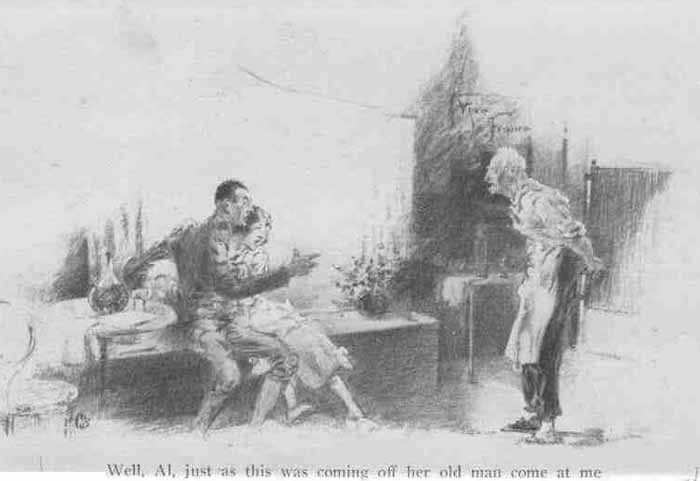The black-and-white sketch depicts a dramatic scene featuring three individuals. On the left, a man and a woman are sitting closely on a bench, her arms wrapped around him, suggesting intimacy. The man, possibly in pajamas, is pointing his finger aggressively at an older man on the right, who is wearing an apron and appears hunched over with a shocked expression on his face. Surrounding them, details emerge: a vase with flowers on the bench, a chair nearby, a wash basin behind the younger man, and possibly a table behind the older man, indicating a domestic setting. The sketch is impressionistic and uses negative space effectively to convey the scene. Underneath the illustration, text reads, “Well Al, just as this was coming off, her old man came at me.” The context of the dialogue is unclear, but it adds a layer of tension and mystery to the image.